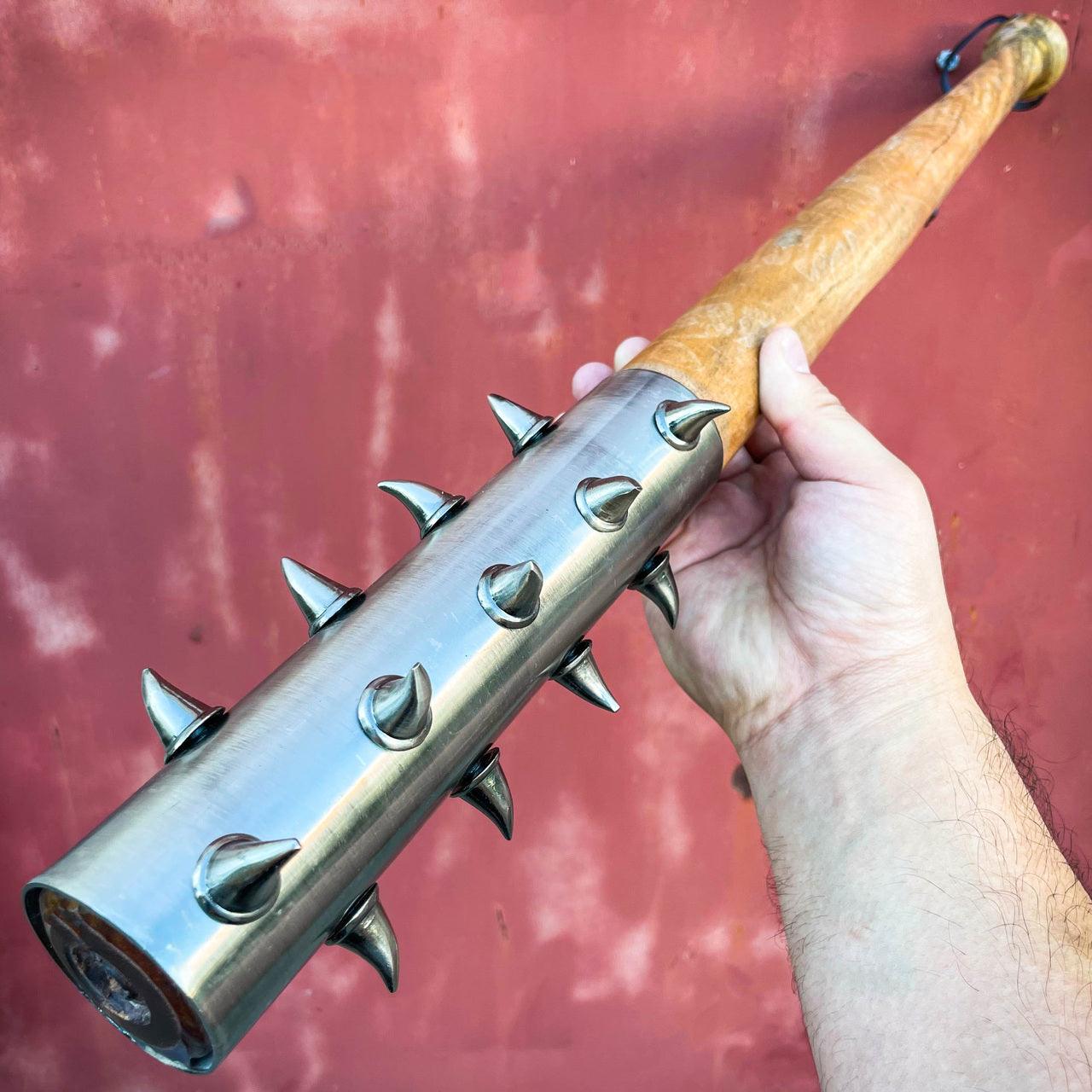In the image, a man's hairy right hand firmly grips the middle of a makeshift weapon resembling a baseball bat. The background is a vivid cherry red, providing stark contrast to the object in focus. The bat, seemingly constructed from wood, maintains its traditional handle in the upper right corner. However, a notable transformation occurs at the tip, where a metal-spiked cylinder envelops a significant portion of the bat, taking up nearly a quarter of its length. The spiked metallic section, resembling steel, is adorned with three rows of substantial, pointed spikes; there are five spikes in the top row, four on the left, and four on the underside, totaling 13 visible spikes. These menacing, thorn-like protrusions, each about two inches long, suggest a weapon designed for considerable impact. The bat also features a lanyard at its foot, situated in the upper right side of the frame, adding to its practical, albeit intimidating, functionality. Overall, the image captures a close-up of the man's forearm and the formidable weapon against the rich red backdrop, emphasizing the juxtaposition of familiar sports equipment repurposed into a fearsome tool.